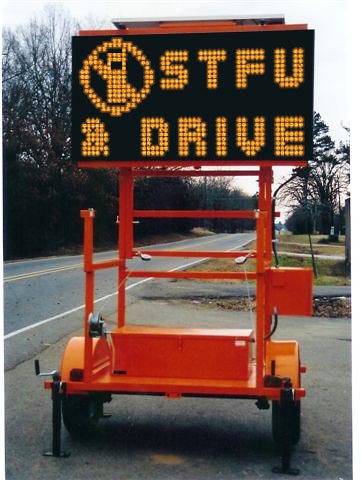This is a photograph taken from the right side of a two-lane road with a double solid yellow line down the middle and white lines on the shoulder. The primary focus is a temporary, mobile digital warning sign mounted on a bright orange, two-wheeled metal structure for easy relocation. The sign features a black background with orange neon-lit text reading "S-T-F-U and DRIVE" and a schematic image of a cell phone with a line drawn through it, indicating a prohibition on cell phone use while driving. The road is flanked by grassy lawns and driveways, with dense trees on the left and a few scattered trees on the right. The background sky is gray.